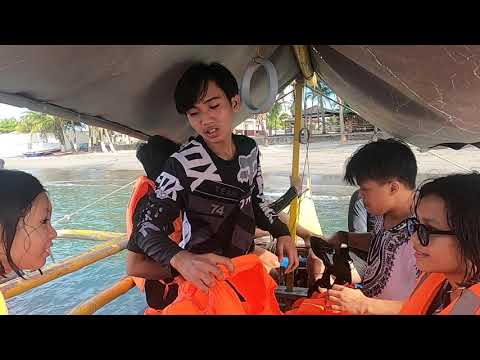The slightly out-of-focus, full-color photograph, enclosed in a black border at the top and bottom, depicts a vibrant scene aboard a long, narrow catamaran, likely situated in a tropical locale such as the Philippines or Thailand. The boat, outfitted with a gray cloth canopy, is constructed from bamboo and features a yellow rail for safety. Inside the vessel, a group of young people with dark hair, including one wearing a shirt with the number 74, sits and stands against the vibrant coastal backdrop. Prominently, a young male stands at the center wearing a black long-sleeved Fox Racing t-shirt, appearing to hand out orange life preservers to his companions. In the background, serene palm trees sway near a beach dotted with straw huts and cabanas, basking under the high-noon sun, as their shadows lie directly beneath them. The lush beach setting with clear indications of tropical flora and humble beachside structures enhances the image's overall atmosphere of leisure and adventure.